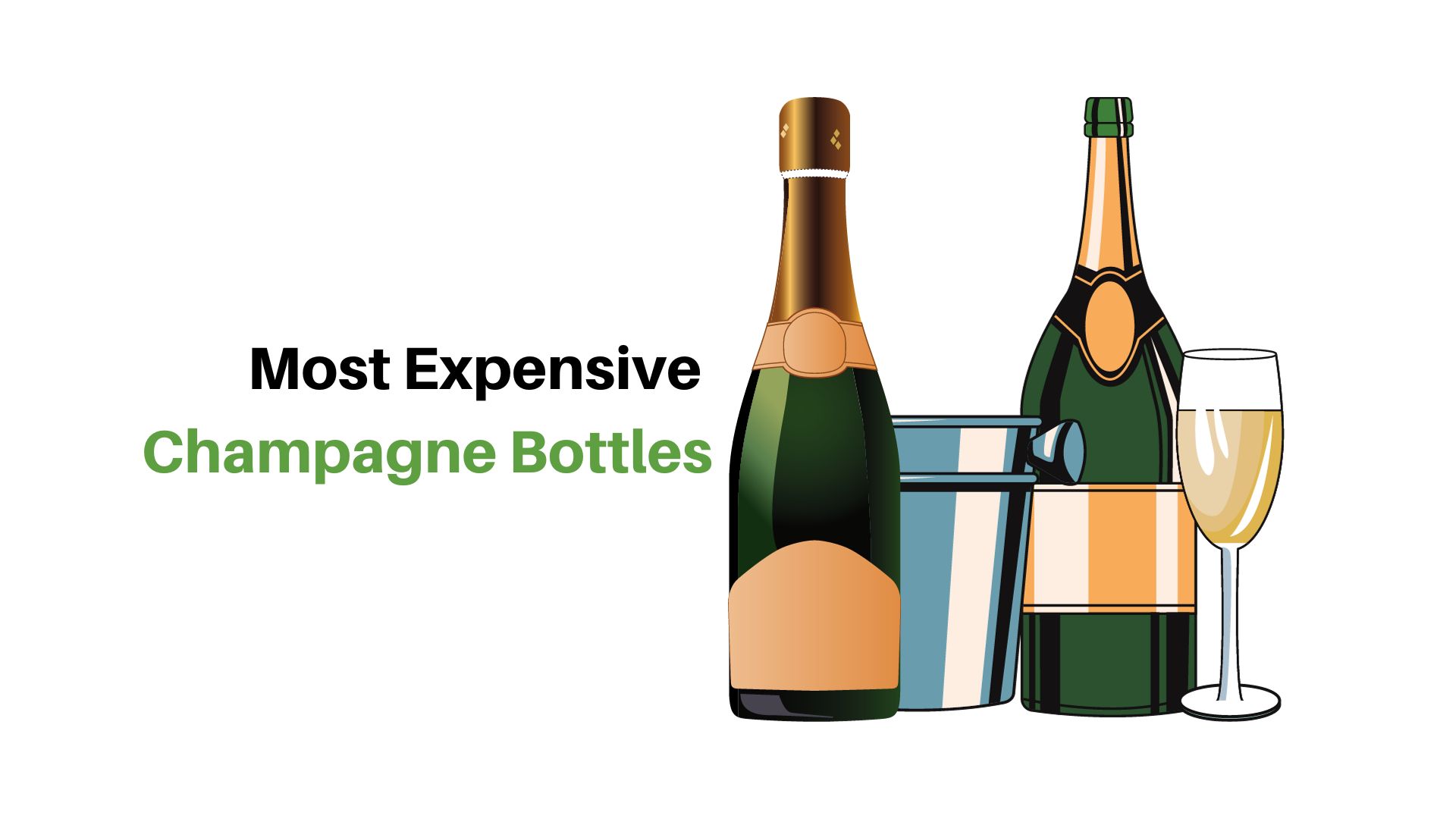This drawing, resembling an advertisement with a cartoonish comic strip style, features two champagne bottles accompanied by a glass and an ice bucket. The left champagne bottle, unopened and wrapped at the top, is very dark green with some brown accents and gold detailing on the label, extending towards the neck in a blue and gold pattern. Partially obscured by this bottle on the right is a second bottle of similar design, which is open and prominently displays a copper-colored label around its neck. Between the two bottles sits a small silver ice bucket, about half the height of the bottles. Positioned further to the right is a flute-shaped champagne glass filled with a yellow liquid, suggesting champagne. Black text above the scene reads "Most expensive," with "champagne bottles" below it in green text, completing the graphical presentation.